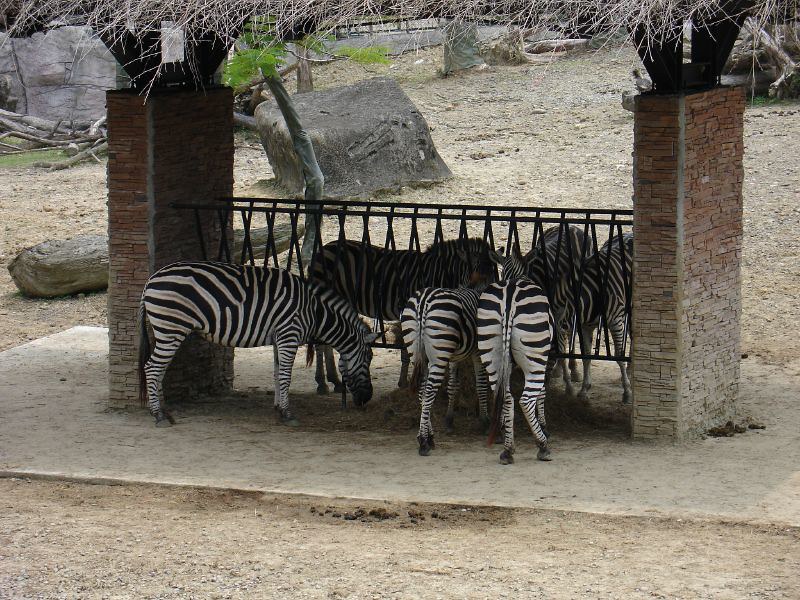The zoo enclosure features six zebras, evenly divided with three on each side, all gathered around a central feeding structure. This feeding area comprises two stone pillars supporting a thatched roof to protect the hay from inclement weather. Suspended between the pillars is a black, crisscrossed metal grate that holds the hay. The enclosure's ground is a mix of light brown dirt, gravel, and sand, with large gray boulders, dead logs, and stumps scattered to simulate a natural habitat. Sparse greenery is visible on the left, and a fence and watering trough can be seen in the background. The zebras, black and white, have their heads down, feeding from the hay beneath the grate. Zebra droppings are noticeable near the right pillar. This well-designed enclosure provides a realistic environment for the zebras while ensuring they have a designated, weather-protected feeding area.